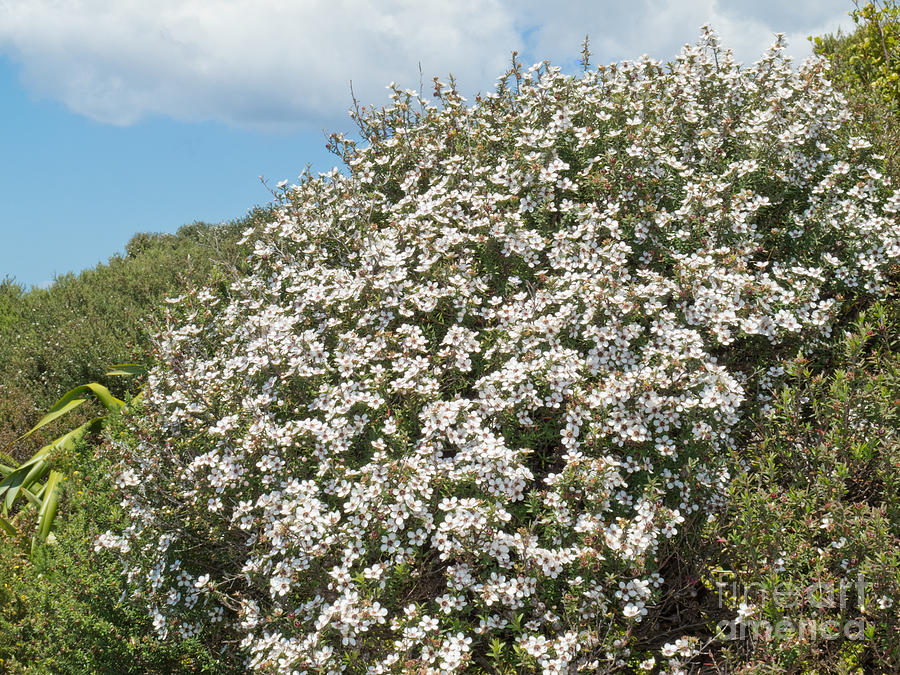The image depicts a vibrant hillside filled with lush, green foliage and abundant flowering shrubs. Dominating the scene is a large, central bush adorned with numerous white flowers, each featuring five petals and a yellow or red center. This bush is surrounded by additional greenery, with smaller shrubs and plants on both sides, including one plant on the left with long, narrow leaves reminiscent of a corn plant. The background reveals a couple of small trees at the hill's summit. Above, the sky is a clear, summer blue dotted with fluffy white clouds, indicating a bright midday. In the lower right corner, the watermark "Fine Art America" is clearly visible. Overall, the landscape is rich with natural details, showcasing a thriving ecosystem on a sunny day.